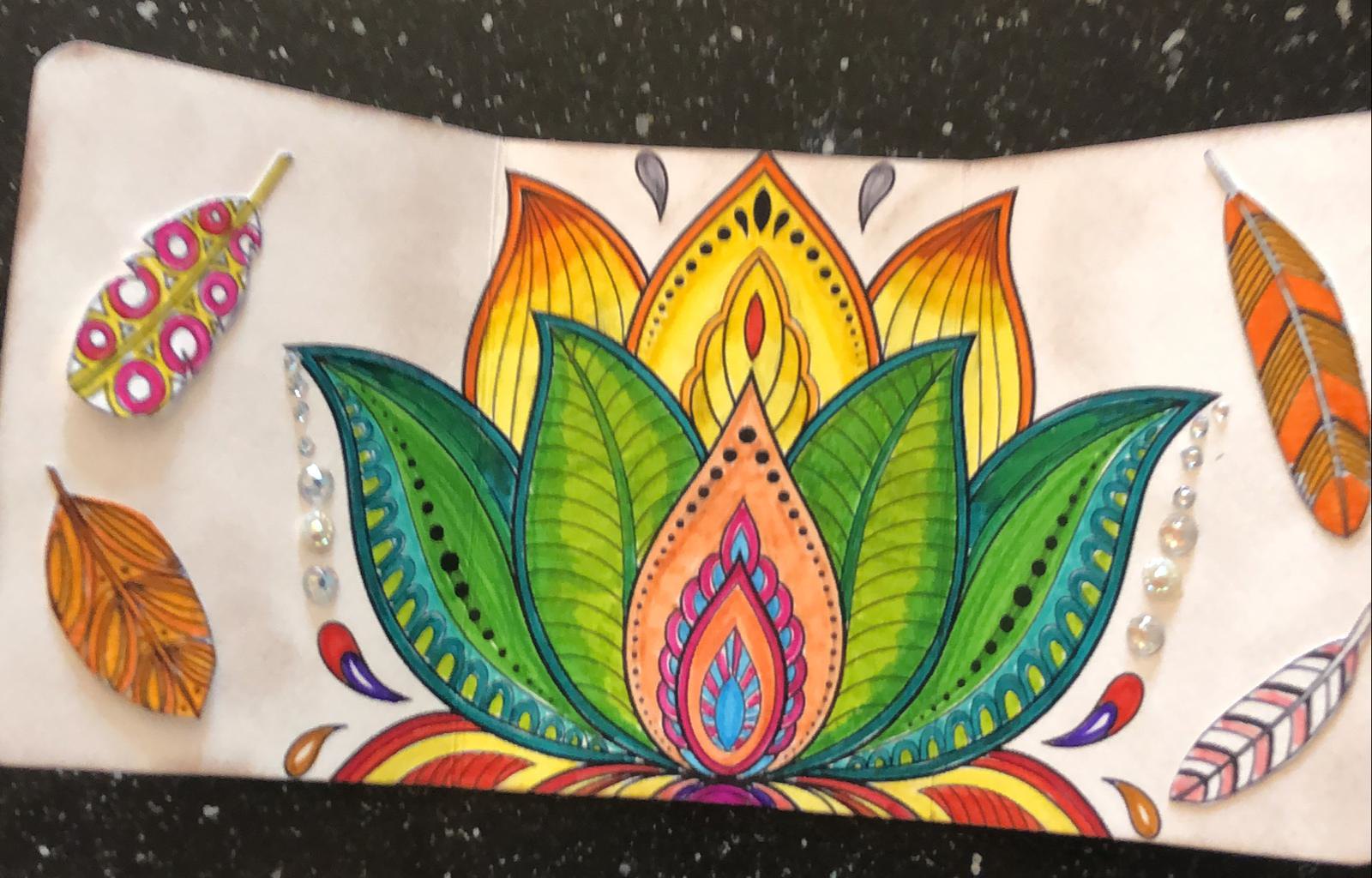The image appears to be a foldable material, possibly a mural, featuring a vibrant and colorful design. The central motif resembles an aloe plant, depicted in a variety of colors, including green, yellow, red, orange, and blue. The plant-like illustration is complemented by intricate patterns.

Above the main plant, there are two gray teardrop shapes, seemingly dyed directly onto the material. The background is a speckled combination of green and gray.

Additionally, the mural includes several pasted or glued images of leaves with distinct colors and patterns:
1. A leaf in beige and brown hues.
2. A leaf with pink dots and white central spots.
3. A leaf with orange and brown stripes.
4. A leaf with pink, white, and black stripes.

The overall composition is dynamic and visually striking, combining both drawn and real elements to create a textured, colorful piece.